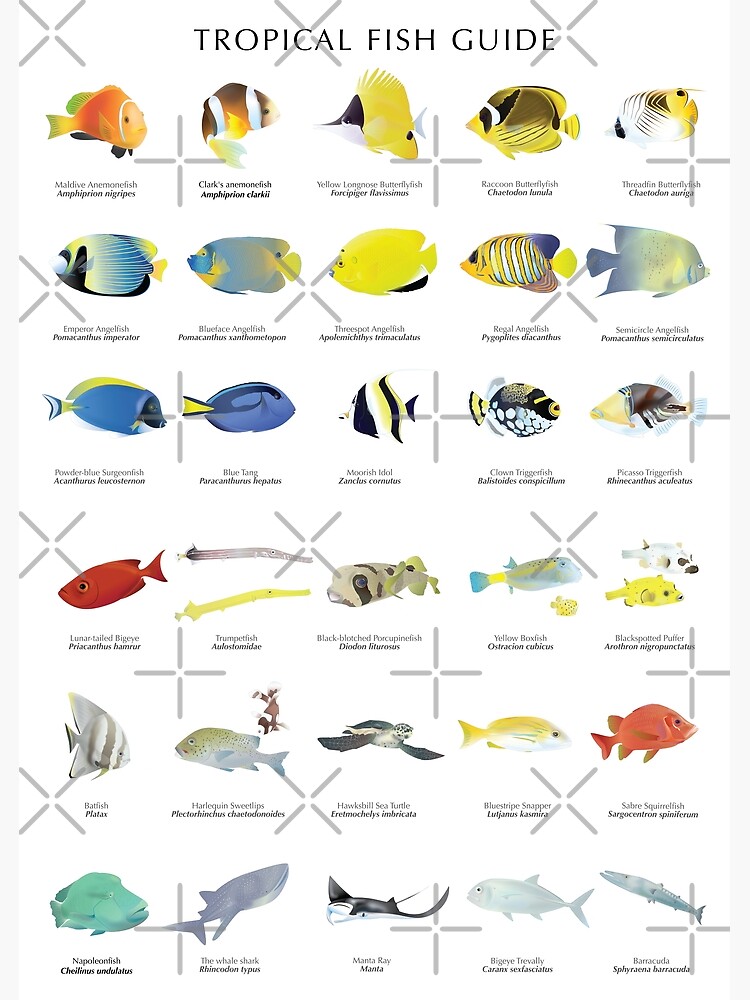The image is a full-color vertical print with digitally added watermarks, specifically rows of X's, to prevent unauthorized copying. The top of the image features the title "Tropical Fish Guide" in bold, capitalized black letters. This guide showcases a diverse array of tropical fish, organized in a grid with six columns and five rows, making a total of thirty fish.

The fish displayed are vibrant and varied. While the text identifying each species is too small to read, the colorful illustrations vividly capture the beauty of these aquatic creatures. The colors range from intense blues and bright yellows to deep reds and silvers. Some of the notable fish include an orange fish with a white stripe and green-yellow fins, a brown fish with white stripes and yellow fins, and an entirely yellow fish with a black tail. Other striking fish include a black, yellow, and white-striped fish, a blue fish with yellow detailing, and an eel-like fish in both gray and yellow. There's also a distinctive red fish, several blue fish with varying patterns, and a turtle with greenish-black coloration. This guide not only highlights the diversity in size and color but also emphasizes the unique patterns of each species, making it an eye-catching and informative piece.